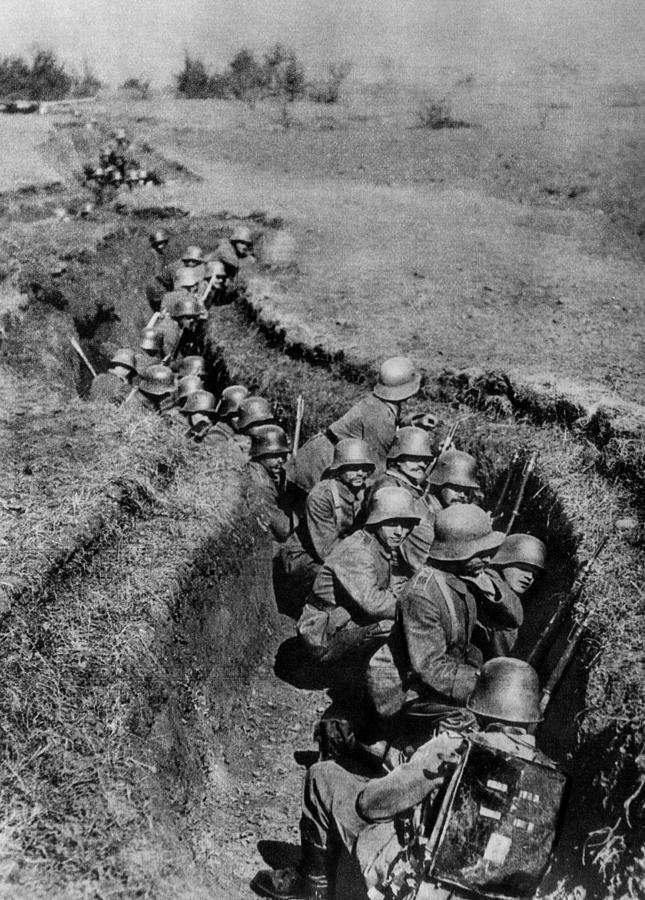This black-and-white photograph from the World War I era depicts a group of German soldiers hunkered down in a long, curved trench that stretches from the center to the left side of the image. The grainy quality of the photo, indicative of its age, enhances the somber atmosphere. The soldiers, numbering a couple of dozen, are captured in various postures—kneeling, crouching, and peeking out, all facing the right side of the image where the enemy is presumably located. They are equipped with rifles, many featuring bayonets, and each wears a distinct rounded helmet tapering at the back, along with backpacks. The scene is stark, with sparse trees visible in the background, and the men’s expressions of discomfort add to the photo’s grim authenticity.